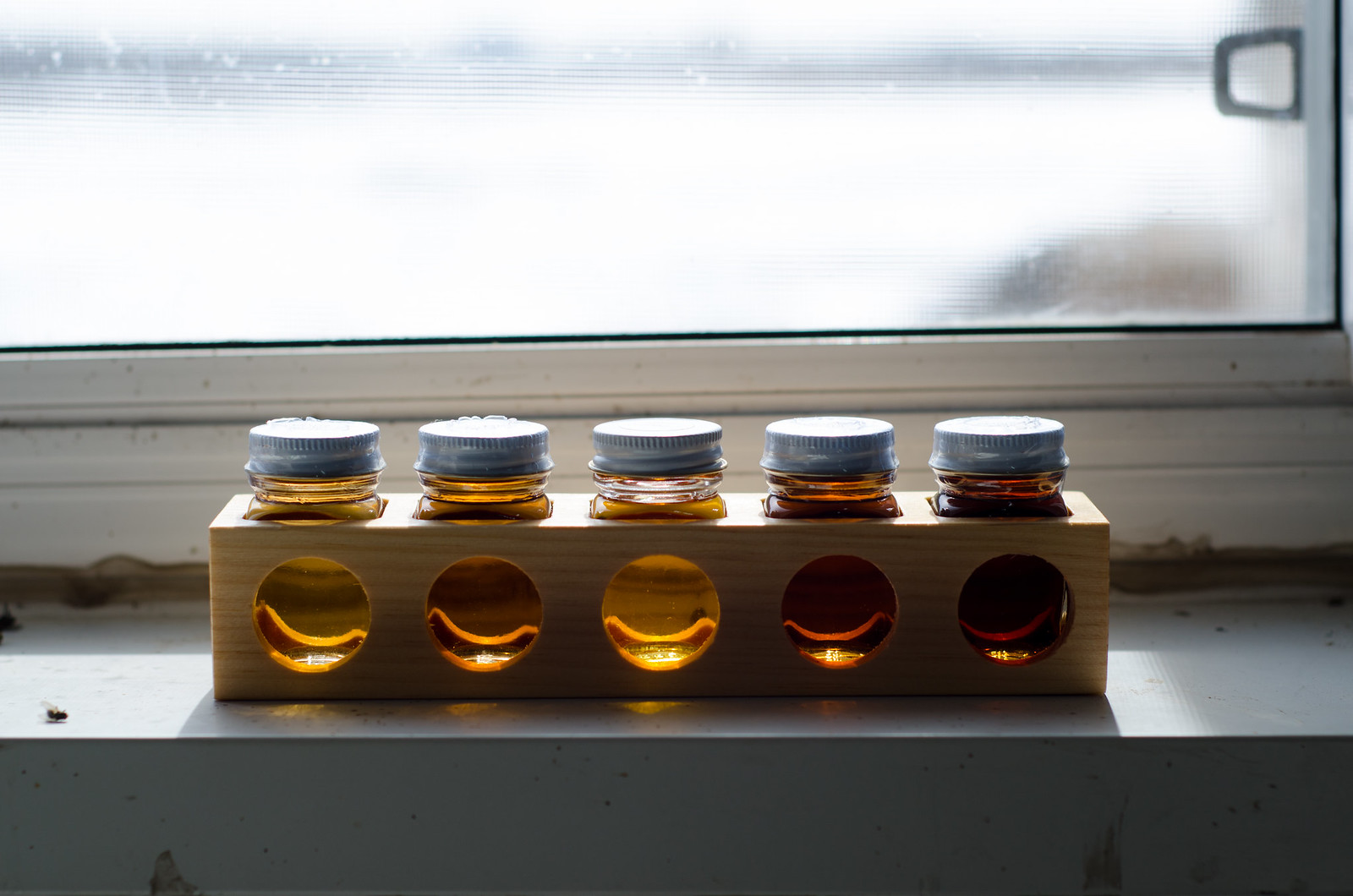This vibrant color photograph captures a rustic scene set against a white windowsill, where a long, rectangular pine wooden box with circular holes punched along its top and sides houses five glass jars filled to the brim with amber-colored honey. The jars, sealed with silvery metal lids, display a gradient of hues from golden yellow to dark amber, suggesting different flavors. The window behind the setup, slightly cloudy, hints at a misty day outside. The bottom of the windowsill is dirt-streaked, and a dead fly, lying on its back with legs upturned, can be observed towards the front left side. The overall image evokes a sense of natural simplicity, with details that emphasize the textures of the wooden box, the clarity of the glass jars, and the subtle dirt and dust on the windowsill.